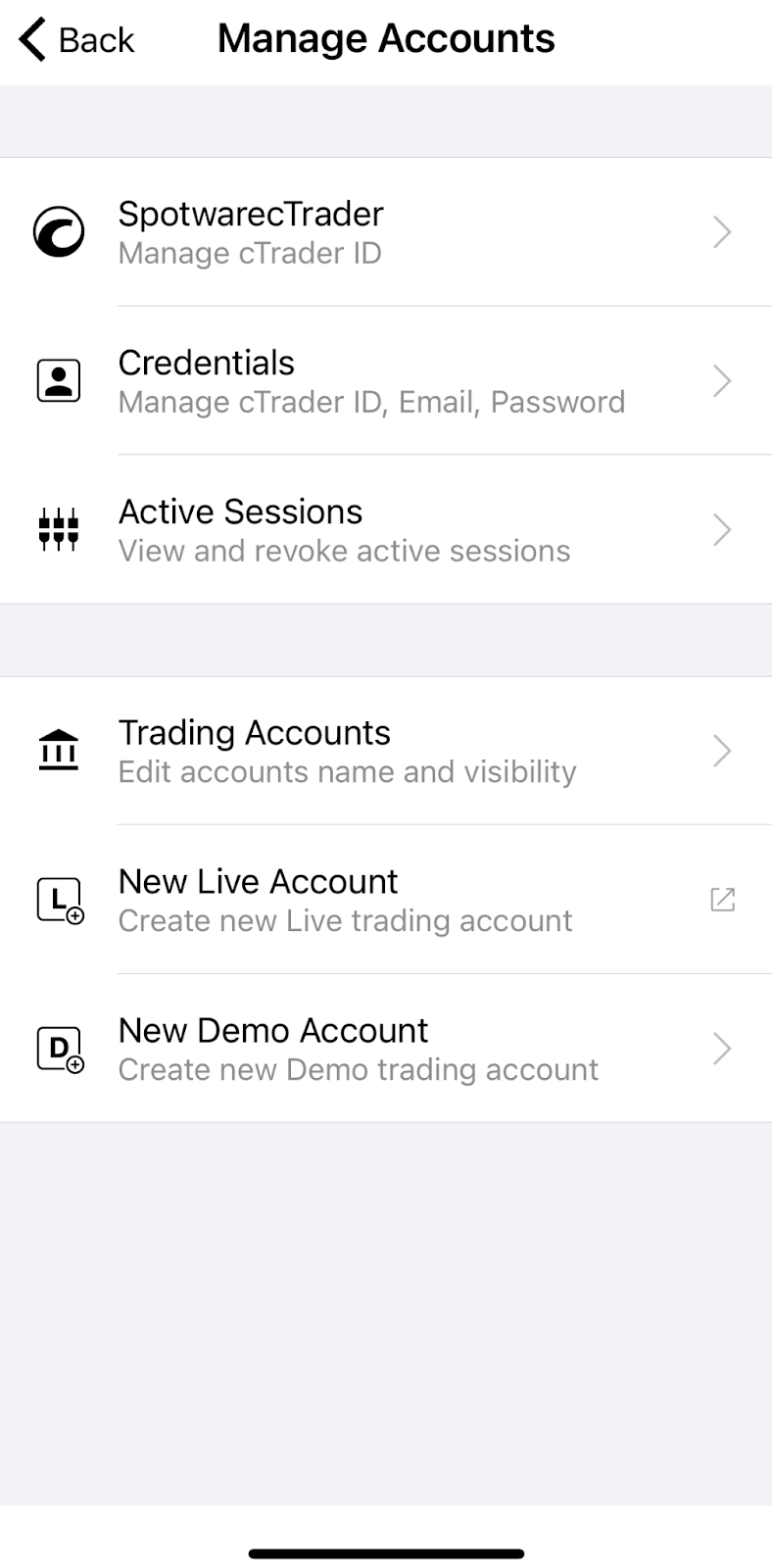This vertical smartphone screenshot depicts a trading account management interface. At the top, "Manage Account" is prominently displayed in the largest font, and a "Back" button with an arrow icon is situated in the upper left corner. Beneath the main heading, it reads "Spotware cTrader" with a subtext "Manage the cTrader ID."

The interface includes a series of options listed vertically from top to bottom:

1. "Credentials" - accompanied by a small icon of a person.
2. "Active Sessions" - featuring a corresponding icon.
3. "Trading Accounts" - with its respective icon.
4. "New Live Account" - marked with an indicative icon.
5. "New Demo Account" - also paired with its unique icon.

On the right side of each listed item, there is an arrow icon suggesting that additional settings or options can be accessed by selecting them.